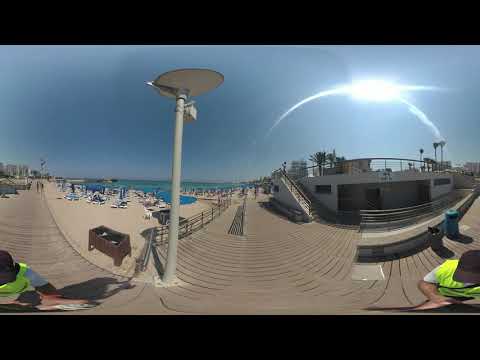The photograph captures a vibrant beach scene during the daytime, taken with a 360-degree camera. Dominated by a clear blue sky, a radiant white sun sits in the top right corner, casting a bright streak across the sky. A prominent gray pole with an oval top stands tall near the center-left. The wooden boardwalk, a rich coffee-brown, spans across the image, with trash cans and possibly a bin for shoes alongside it. On the bottom left and right corners, a man wearing a high-visibility lime green vest, a white t-shirt, and a black baseball cap, holds the 360-degree camera. To the left, the walkway transitions into a sandy beach, teeming with people relaxing under blue sunbeds and umbrellas. The light beige sand meets the teal ocean waters at the beach's edge. In the background, a city skyline rises to the left, while the right side of the image features a gray and white building with a staircase and black railings. Beyond and above this structure, silver railings decorate the outdoor space. The scene is tranquil, epitomizing a bustling yet serene day by the seaside.